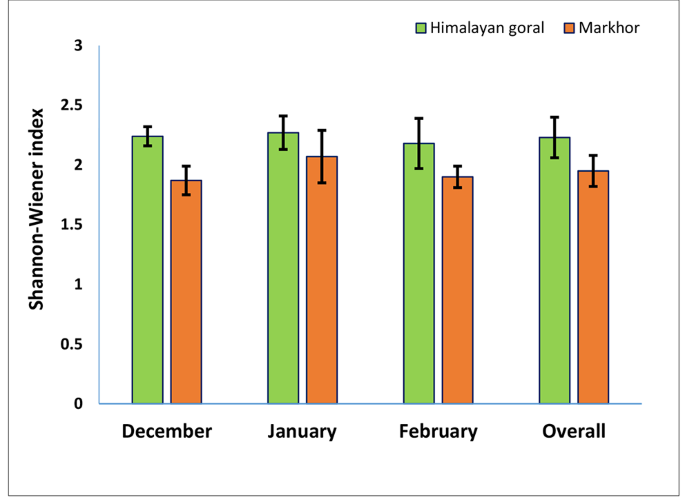This is a detailed graph depicting the Shannon-Wiener Index. The graph features green and orange bars representing the Himalayan Goral and Markhor, respectively. The text to the left of the graph reads "Shannon-Wiener Index," with a numerical scale ranging from 0 to 3 in increments of 0.5. The x-axis denotes the months December, January, February, and an overall category. The top right corner specifies the legend, with the green color identifying the Himalayan Goral and orange identifying the Markhor. 

For each month and the overall category, the green bars for the Himalayan Goral consistently register slightly higher values than the orange bars representing Markhor. In December, the Himalayan Goral reaches approximately 2.25, while the Markhor is just under 2. In January, the Himalayan Goral again hovers around 2.25, with the Markhor close to 2. This pattern continues across February and the overall category, where the Himalayan Goral consistently maintains a marginally higher position on the index. The black text on the chart is clear and the entire graph is neatly enclosed within a rectangular box, making it a typical example of a scientific graph seen in textbooks or academic presentations.